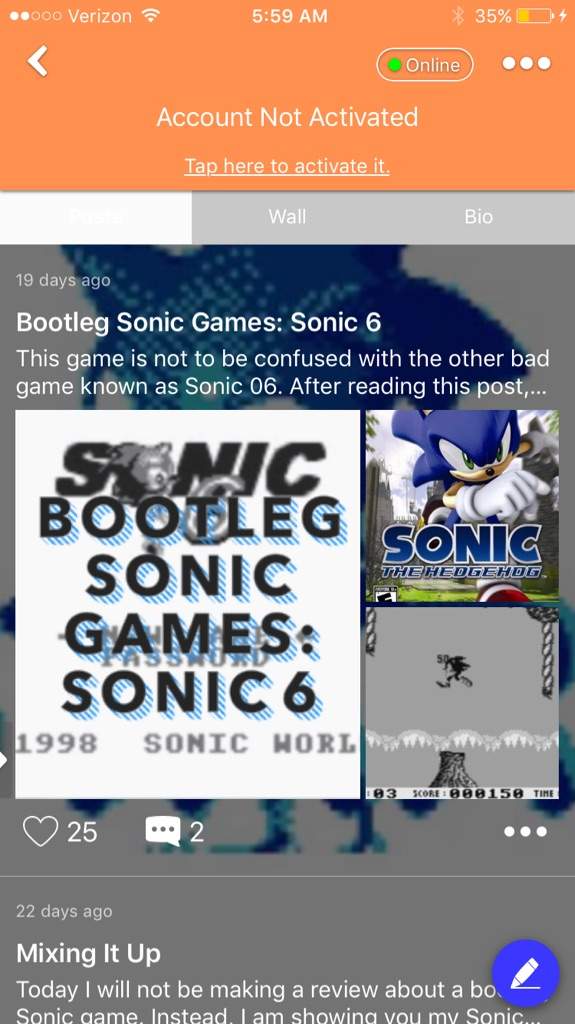The image is a detailed screenshot of a cell phone screen displaying various pieces of information and app interfaces. 

In the top left corner, the Verizon logo is visible. The signal strength is shown as two bars and the Wi-Fi icon is also displayed. The time is centrally located, reading "5:59 a.m." To the top right, a battery icon indicates a charge of 35%.

Directly beneath the status bar, there is a green dot labeled "Online." Below this notification, it reads, "Account not activated. Tap here to activate," with the instruction underlined for emphasis.

Following this, there are two tabs labeled "Wall" and "Bio." Underneath these tabs is a post timestamped "19 days ago" with the title "Bootleg Sonic games: Sonic 6." The post clarifies, “This game is not to be confused with the other bad game known as Sonic ‘06. After reading this post...”

To the left side of this post, there is a white rectangular section which reads, "Sonic bootleg Sonic games Sonic 6 1998 Sonic World." On the right side, there is an icon depicting the blue Sonic the Hedgehog character, facing forward and wearing white gloves. Below Sonic’s image, it says "Sonic the Hedgehog."

Further down, there is another icon that seems to be a screenshot from a game. It shows a character in midair over a volcano, with a game score of "150" displayed. Below this image, there is a heart icon followed by the number "25" and a message icon followed by the number "2."

Overall, the screenshot captures a blend of device status indicators, app notifications, and a post related to a bootleg Sonic the Hedgehog game.